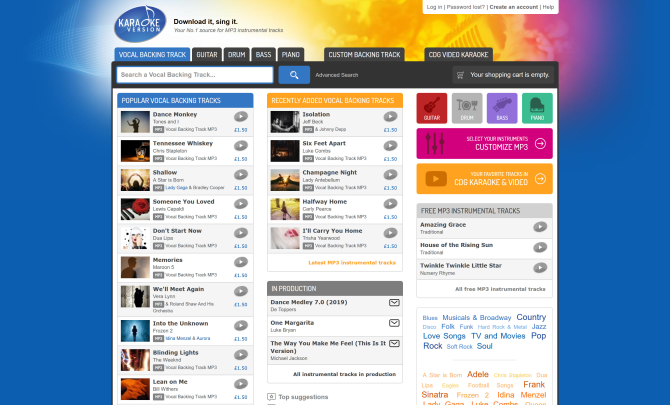The screenshot depicts the main interface of a karaoke app with a visually appealing and user-friendly design. The background is primarily blue, with a colorful, faded image of a microphone behind the main menu options, creating an engaging and dynamic atmosphere.

At the top of the interface, there are several tabbed options for different instrumental backing tracks, including vocals, guitar, drums, bass, piano, and more, allowing users to customize their singing experience. Below these tabs, a prominent search bar invites users to look up their favorite songs or artists.

The main content area features three distinct columns set against a white background. The left column lists popular vocal tracks, providing a quick selection of trending songs. The middle column, highlighted with a blue background, also displays popular vocal tracks, emphasizing their popularity and easy access. On the right, the column is dedicated to recently added vocal backing tracks, showcasing the latest additions to the app’s library.

To the far right of the interface, there is a collection of buttons and menus in various colors—red, gray, purple, and green—most likely representing options for different instrumental tracks such as guitar and drums. A larger red button for customization stands out near the bottom of this column, offering users the ability to fine-tune their karaoke experience. Additional buttons are arranged below to complete the right-hand side of the interface, enhancing the overall navigability and interactivity of the app.